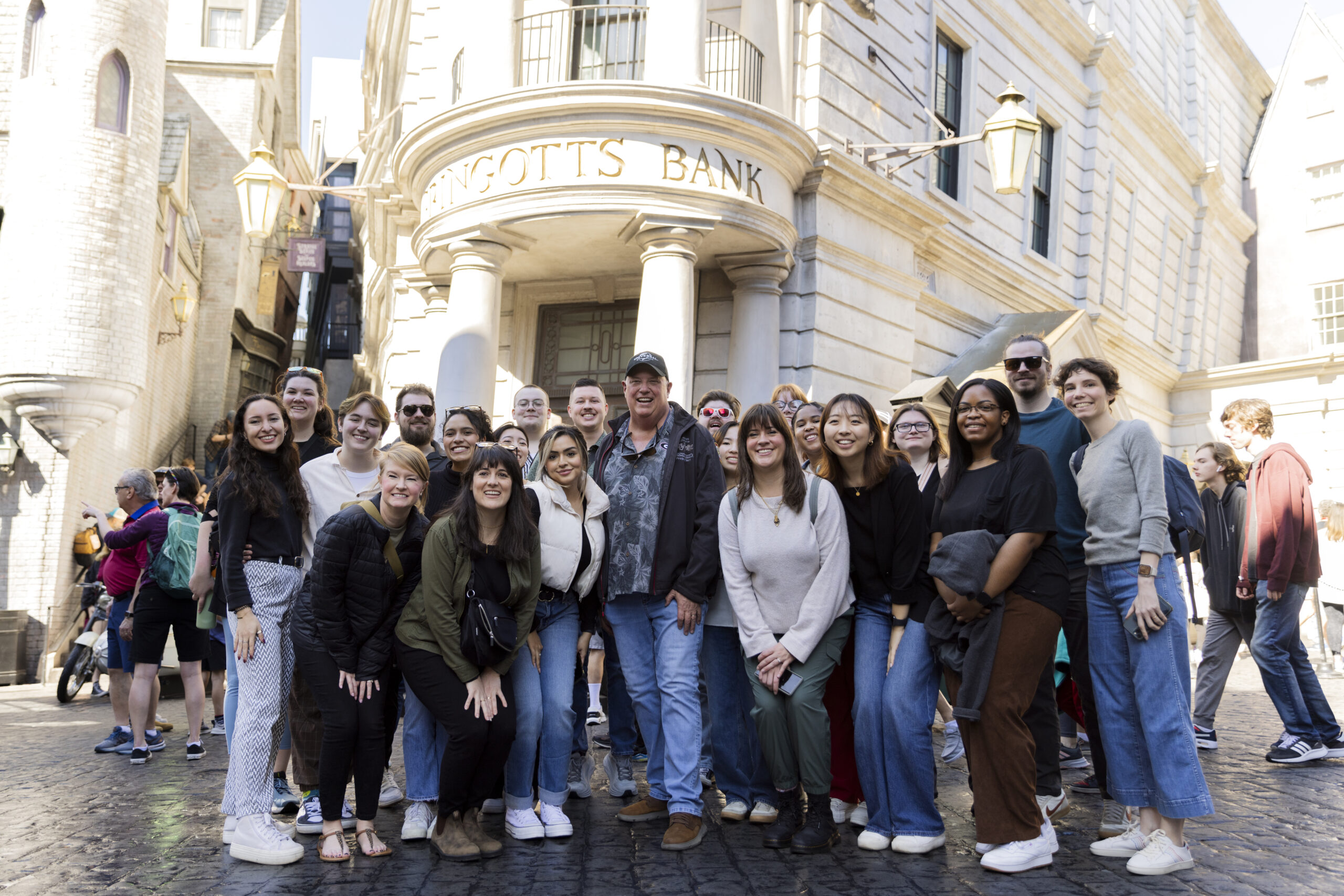In the image, a diverse and large group of men and women, ranging in age from around 25 to 50, are posing and smiling in front of a cream-white, Renaissance-style building with four prominent pillars. The building is designed to resemble Gringotts Bank from the Harry Potter series and is likely part of a replica set at an amusement park, possibly Universal Studios. The front row of women is crouched slightly to ensure everyone in the group can be seen. The façade of the bank features gold lettering, although some of the letters on the right are not fully visible. On the left side of the image, there’s a motorbike and additional people in the background, who are walking and pointing at something off-screen. The group appears bundled up in jackets and long-sleeve shirts, indicating a colder season despite the presence of sunlight.